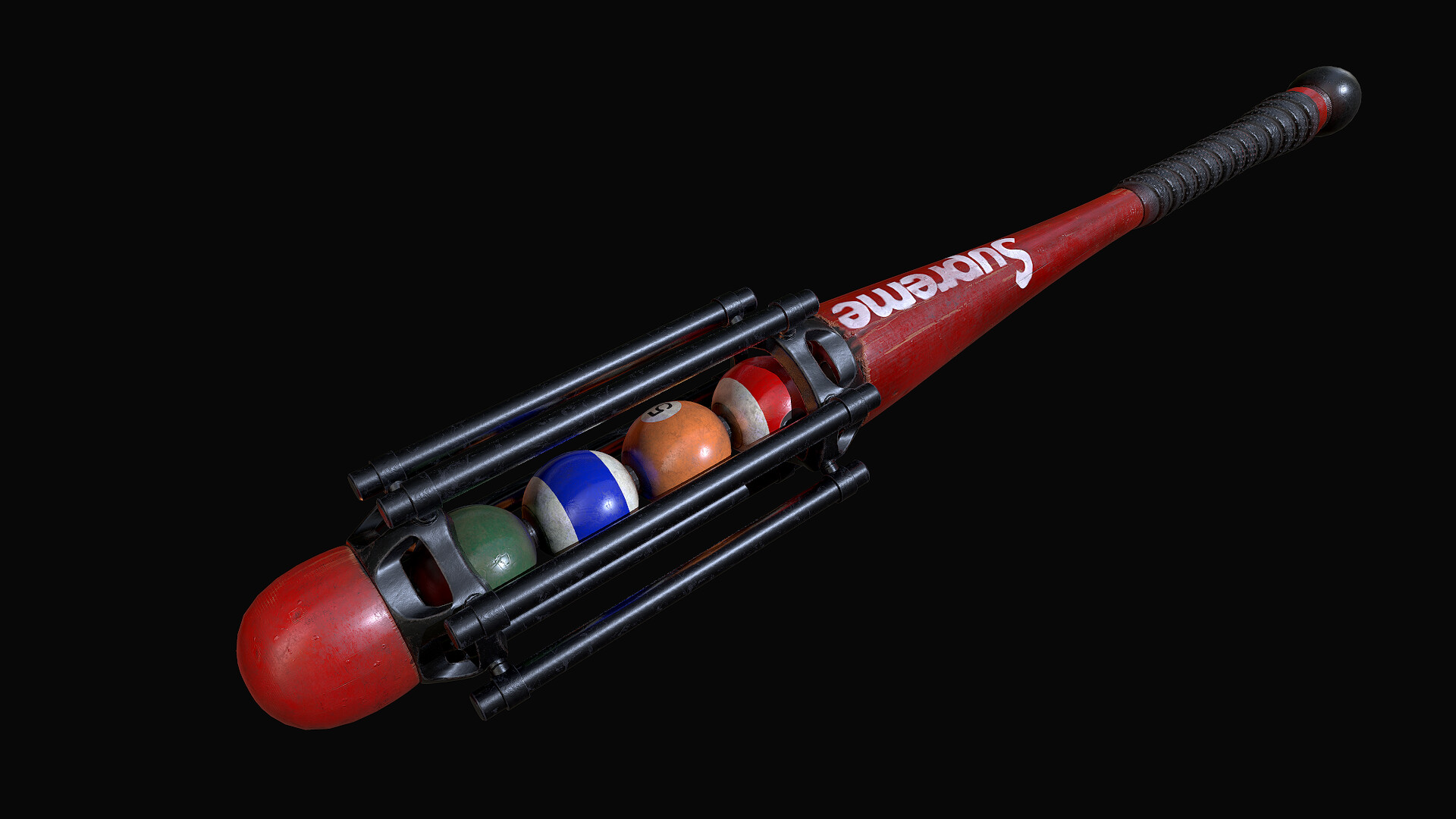The image features a distinctive red baseball bat set against a stark black background. The bat has a black grip and features white lettering spelling "S-U-A-R-E-M-E," although the orientation of the text appears upside down. The bat's interior is hollowed out and holds a collection of four billiard balls, specifically a white ball with a red stripe, an orange ball, a white ball with a blue stripe, and a green ball. A red domed tip caps the end of the bat, and a black plastic contraption secures the billiard balls in the middle. The unusual composition of the bat and balls creates an intriguing visual, with the cue balls’ arrangement emphasizing both solid and striped designs.